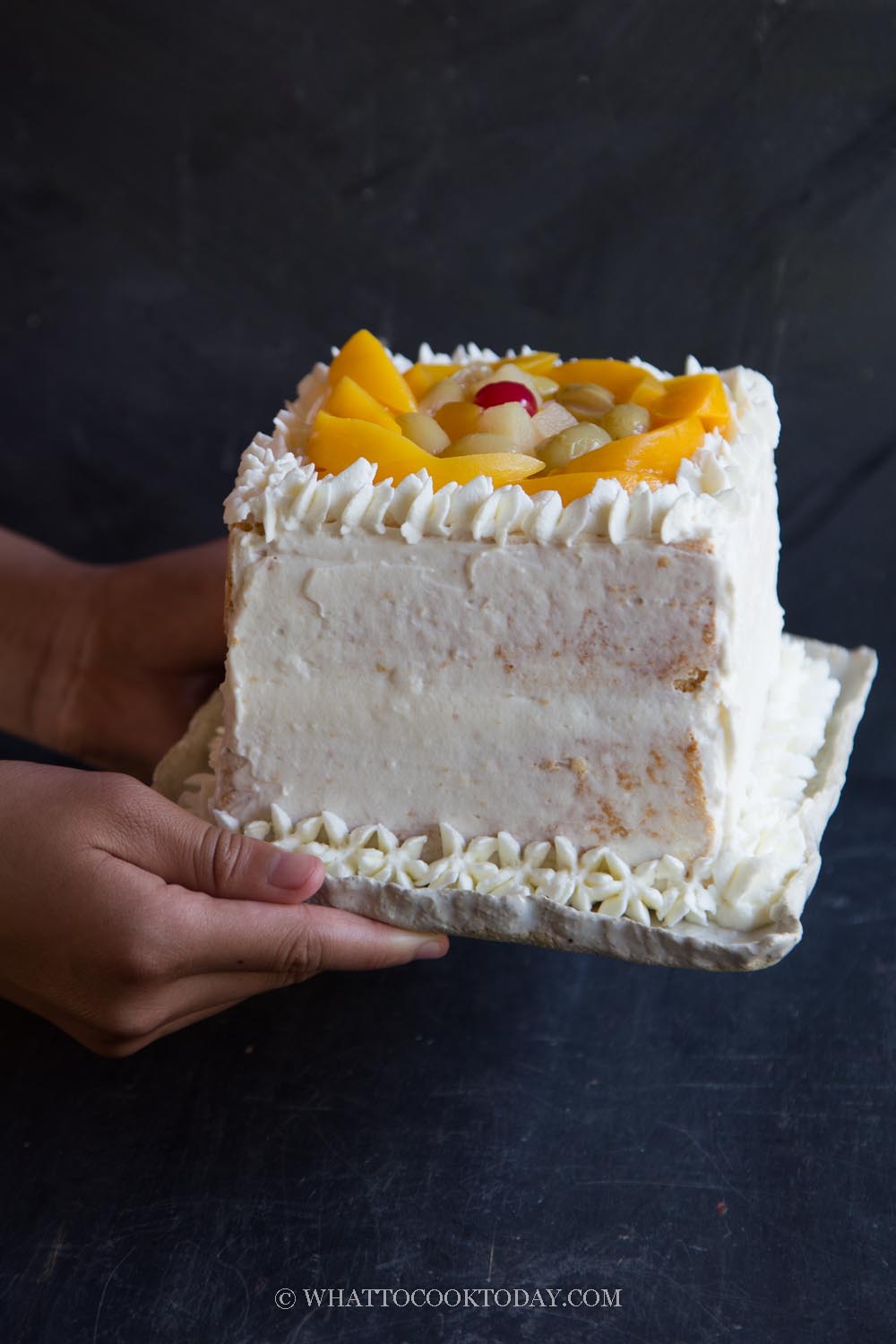This is a color photograph of a small, square two-layer cake held by two hands on an irregularly shaped, white marble-like plate. The cake, approximately four inches on each side, is covered in a thin layer of white or off-white buttercream frosting, through which some yellow cake crumb is visible. The frosting is piped in star and frilly patterns around the base and the top edges. Atop the cake sits an arrangement of sliced fruit forming a circular bed, featuring peaches, grapes, pieces of pear, and a cherry in the middle. The background is a textured, dark blue or almost black color, adding contrast to the image. The photograph includes the watermark "whattocooktoday.com" at the bottom, indicating its source.